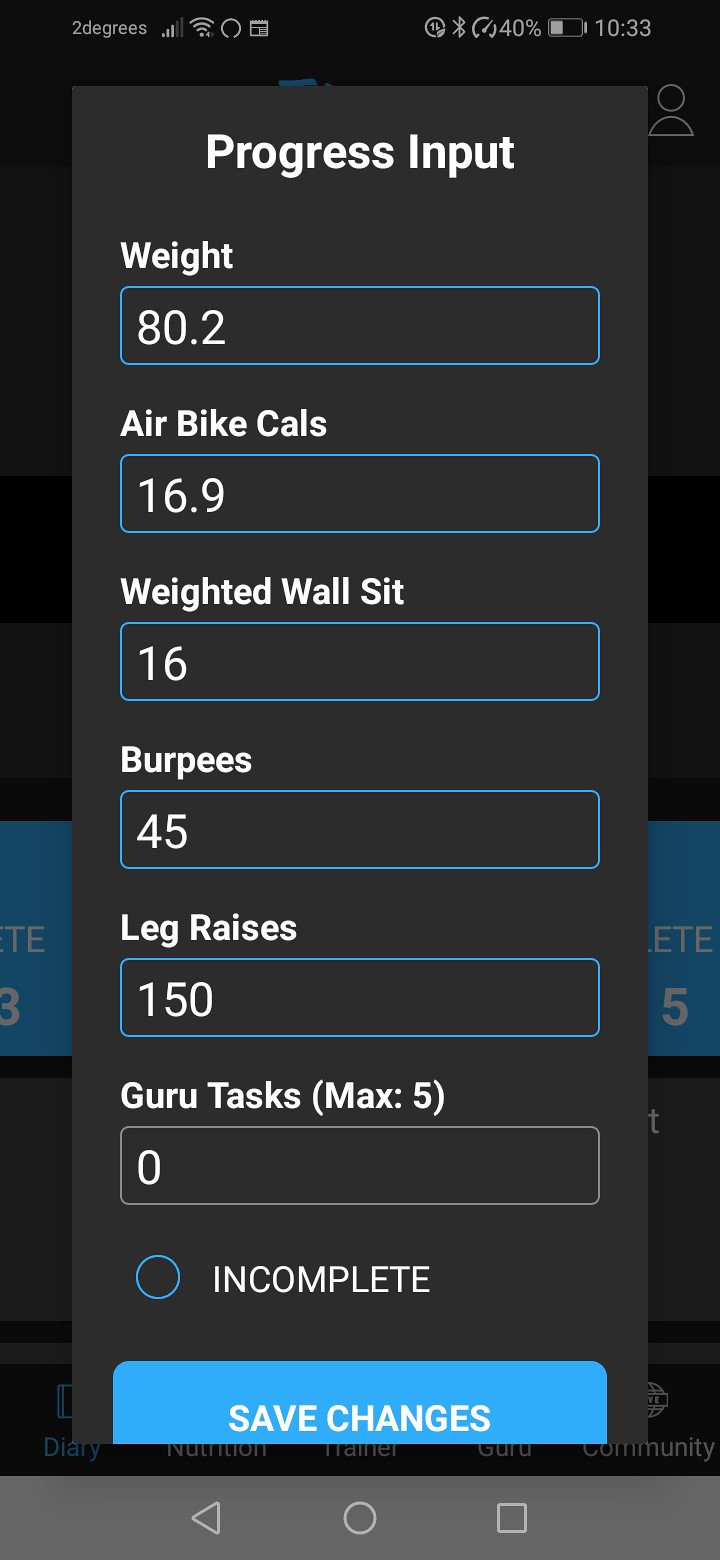This image depicts a screenshot of an exercise app in dark mode on an Android phone, displaying progress inputs for various fitness activities. At the top of the screen, it shows the current time as 10:33 and the battery level at 40%, along with a Bluetooth symbol. The temperature in the top left corner reads 2 degrees. Below these indicators, the app lists several exercise categories under "Progress Input" with details as follows: weight at 80.2 kg, air bike calories at 16.9, weighted wall sits at 16, burpees at 45, and leg raises at 150. There is also a section for "guru tasks" (max: 5), which currently shows 0 tasks completed. An incomplete status is indicated by an empty blue circle, and at the bottom of the screen, there's a blue oblong rectangular button labeled "Save Changes." All text boxes for input data are outlined in a blue border that matches this bottom button.